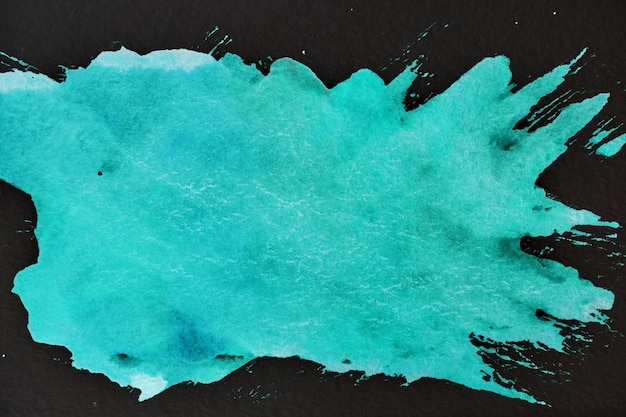The digital image features a smooth, solid black background with a striking, irregularly shaped splash of teal paint dominating the landscape-oriented frame. This vibrant teal, gradient in nature, transitions from darker shades in the bottom left to a purer teal hue throughout. The main splash, reminiscent of an accidental splat of aquamarine-greenish-blue paint, is centered but extends unevenly across the canvas, stretching towards the right, bottom, and top edges with streaks and splashes of color. Upon closer inspection, the teal blob reveals intricately detailed textures resembling scales, accentuated by fine white lines and cracks. Additional darker blue and black elements are interspersed within the teal, along with more prominent white accents along the upper left edge and the tips of the protruding shapes. The image is intriguingly detailed, blending chaotic splashes with subtle, vein-like white lines to create a visually engaging effect.